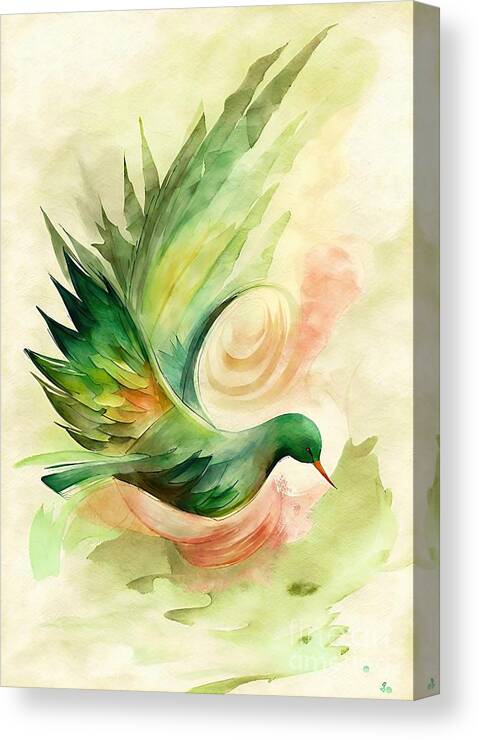This image features a captivating watercolor painting on a canvas, slightly turned to reveal its right side and subtle shadow. A predominantly green bird, with both dark and light green feathery hues, dominates the composition. The bird, captured mid-flight, has a striking reddish-orange beak and an array of elaborate tail feathers accented with streaks of yellow and orange. An intricate spiral emerges from its tail feathers, adding a dynamic sense of movement and depth. The bird’s underbelly or possibly the surface it perches on is tinted with a coral-like, washed-out red, seamlessly blending into the surrounding greenery, which might represent grass or a tree. The background is a delicate mix of ivory, pink, and lighter shades of white and green, enhancing the vividness of the bird. At the bottom right corner, a small reddish design and an indistinct watermark are faintly visible, completing this mesmerizing artwork.